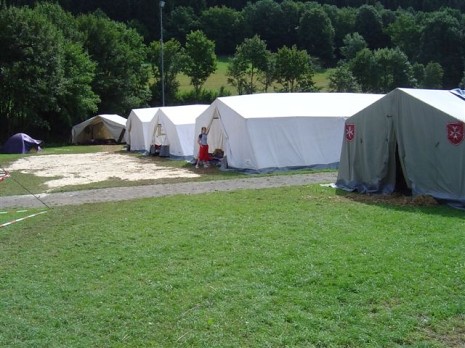In the image, we see a grassy field with a path cutting horizontally through the middle, slightly off center to the right. Positioned from the middle towards the left of the frame are a series of large, long tents, appearing to be medical or army tents. The rightmost tent is dark gray, while the others are white. A man in a t-shirt stands outside the second tent from the right. In front of the third white tent on the left, there's a standard two-person tent, and at the end of the lineup, a tent large enough for five people is visible. The background is dense with trees, adding to the field's secluded feel.